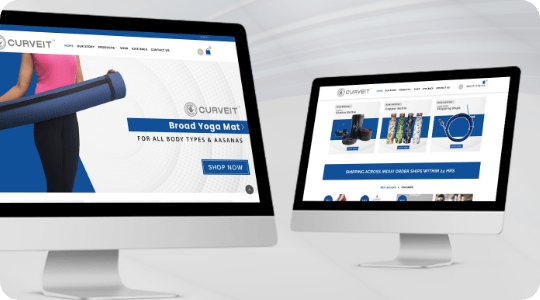This image captures a screenshot depicting a dual-monitor setup, framed against a gray, brushstroke-like background at the top. The monitors, with potentially white or gray exteriors, are mounted on thin metal L-shaped stands. These stands provide support by extending wide at the base and then curving up into the back of each monitor. Both monitors feature black outlines around their screens.

On the left monitor, the website "Curvit" is displayed, evident from the partial logo seen at the top. The Curvit website shows navigation options like "Home," "Our Story," and "Products." Below these options, there is a large image of a woman holding a yoga mat. The woman is dressed in a pink sleeveless shirt and navy blue spandex pants, holding a blue yoga mat with a black carrying strap. The background behind her is a bright cyan on the left, transitioning diagonally into a gray area on the right with radiating gray circles. The webpage also includes text such as the Curvit logo, and descriptions like "Broad Yoga Mat, for all body types and Asanas," with a "Shop Now" button. Beneath these elements is an unclear black circle.

The right monitor also displays the Curvit website, consistent with the navigation options shown on the left monitor. However, this screen highlights three distinct product images: on the left, a coffee maker; in the middle, four patterned sports bottles; and on the right, a coiled cable with exposed ends. Each product image has associated blue order buttons beneath them. Below these products, a larger blue box spans the width of the screen, followed by a combination of blue and black text. The very top portions of four additional images can be seen at the bottom of the page.